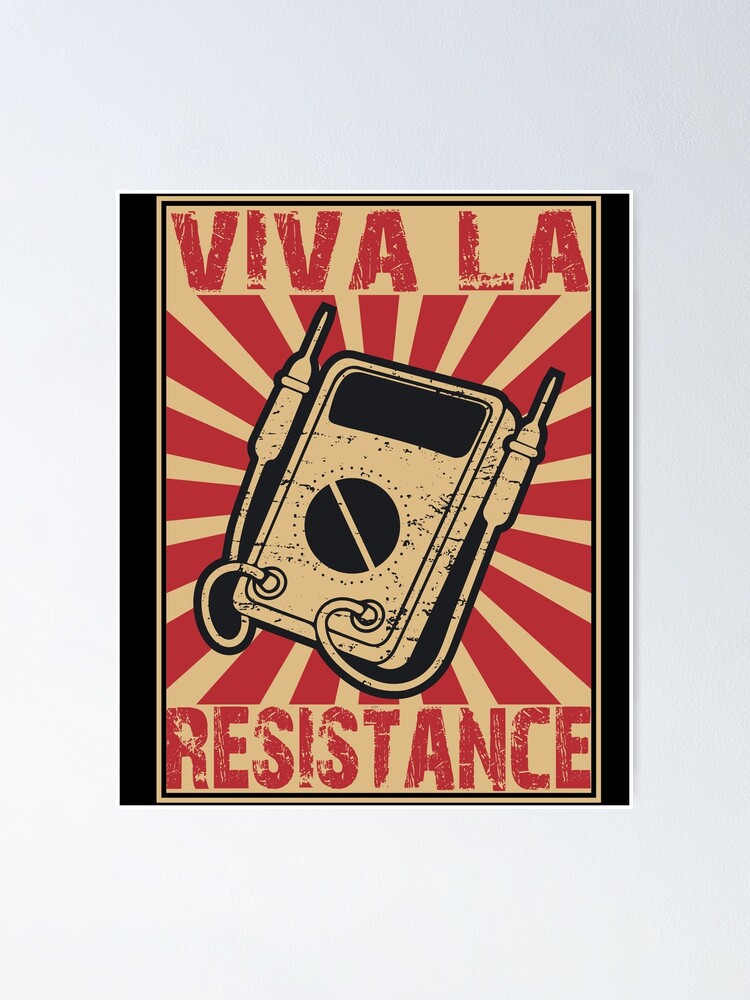The image shows an ad poster with a solid gray background. The poster itself is bordered by vertical black lines on both the left and right sides, framing an off-white, beige center. Across the top and bottom, bold red text declares "Viva La Resistance." The central design features a sketch-like illustration in the same beige and black tones, depicting a rectangular device with a horizontal black display line at the top. At its center, a black circle marked by an angled line suggests a turnable knob. From both sides of this circular control, pointed probes emerge, each connected to the device by wires. Radiating outward from the device are large red rays, adding a dynamic, sunburst effect that matches the vibrant red lettering. The overall impression is one of a call to action, seemingly promoting a rebellion or resistance, although no specific details or dates are provided.